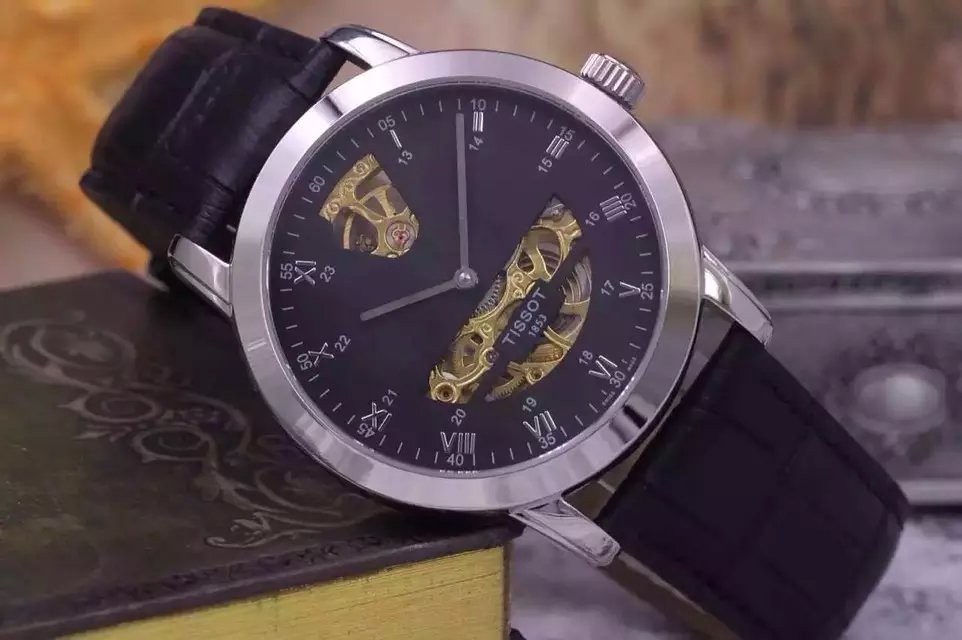This photograph captures a sleek wristwatch, elegantly propped against a book. The watch features a sophisticated black strap made of supple leather. Its watch face is a striking contrast of stainless steel silver, encasing a deep black dial. The dial is adorned with refined silver Roman numerals marking the hours, instilling a classical charm. Additionally, the perimeter of the watch face is detailed with minute markers that range from 0 to 60, enhancing its functionality and precision. The combination of timeless Roman numerals and practical minute indicators creates a perfect blend of style and utility.